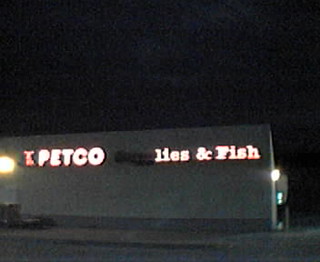In this nighttime or early morning image, a Petco store stands illuminated against the dark sky. The exterior of the building is predominantly white, transitioning to gray at the base. A gray sidewalk stretches in front of the store. On the left side of the store's facade, there's a round light fixture mounted on the wall. The store's name, "Petco," is prominently displayed in vibrant red letters. However, the neon lighting is partially malfunctioning; the word "supplies" is only partially illuminated, leaving "L-I-E-S" visible, while the rest of the letters remain dark. To the right of the Petco sign, a red neon outline of a dog is clearly visible, maintaining its bright glow despite the other lighting issues.